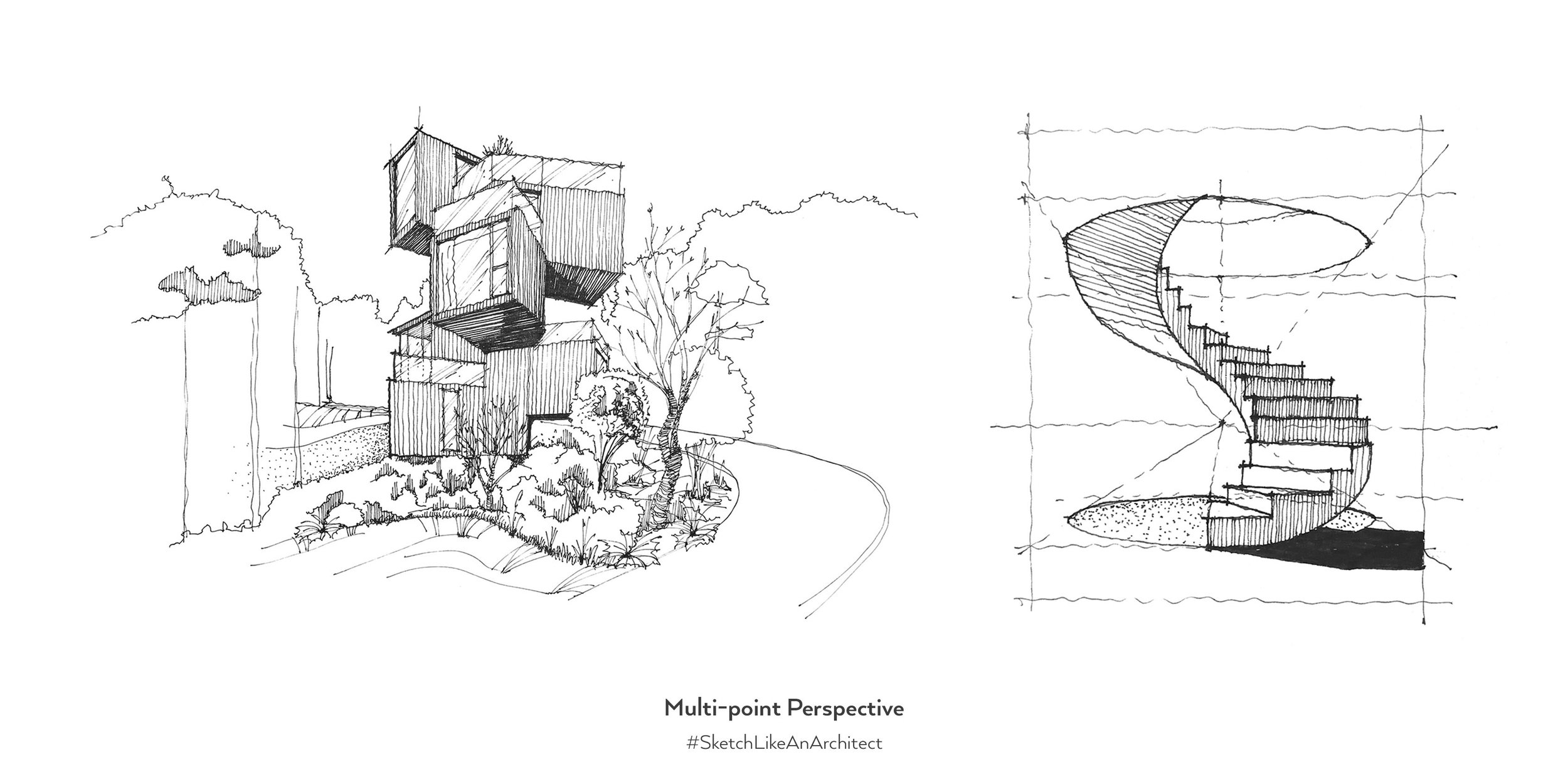This image features two intricate architectural sketches, each illustrating a unique concept in multi-point perspective, emphasized by the caption "multi-point perspective" and the hashtag "#sketchlikanarchtect" at the bottom.

On the left side of the image, there is a highly modern house design composed of several cubic structures stacked and arranged at various angles. The house showcases four distinct levels, each adorned with large floor-to-ceiling windows. Most levels feature glass railings, suggesting roof and observation decks, giving the structure an innovative and open feel. The house is set against a natural backdrop, with trees and bushes providing a contrasting serene environment.

On the right side, the image displays a sophisticated freestanding spiral staircase, meticulously sketched with precise lines that one might find in an architect's or engineer’s detailed drawing. The stairway spirals upwards from a circular base, rising elegantly within a framework of grid lines that reinforce the perspective. This, combined with two diagonal lines converging at the vanishing point, exemplifies advanced architectural drawing techniques.

Both sketches are rendered in either pencil or pen, contributing to a cohesive and detailed study in architectural artistry and perspective.